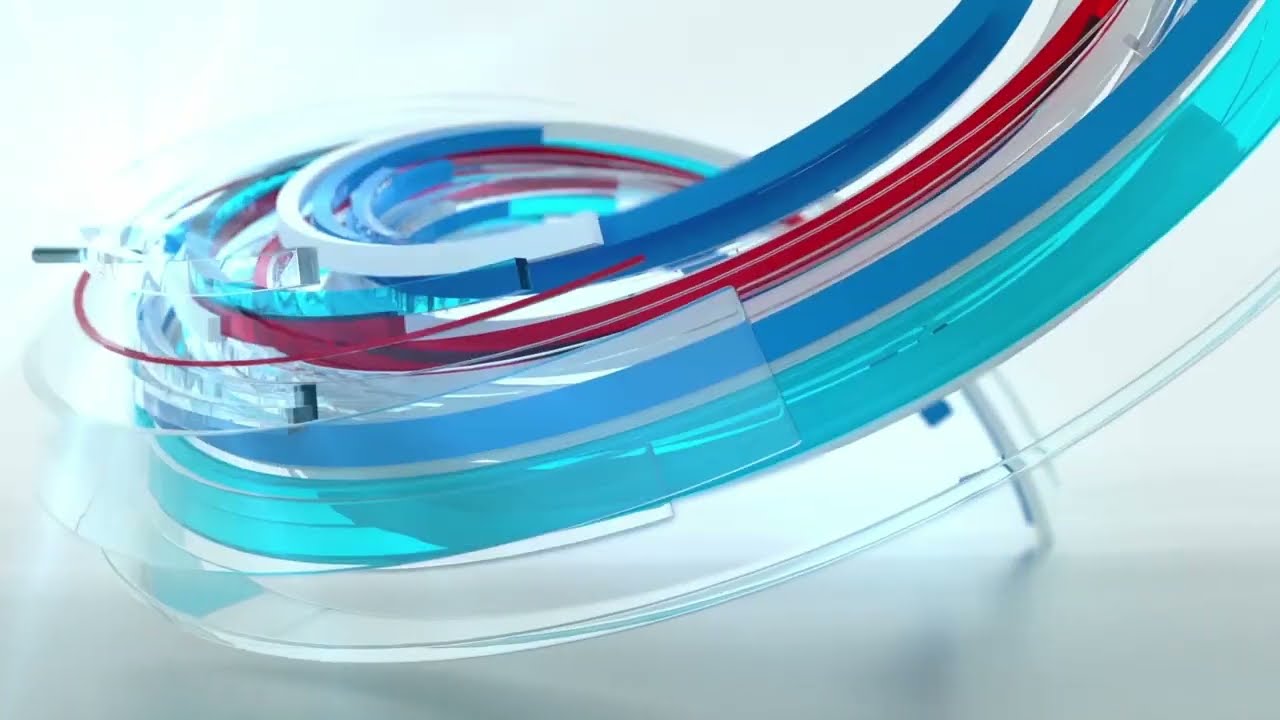The image showcases a 3D-rendered, modernist plastic sculpture that gracefully swirls from the upper right to the lower left before curving back behind towards the lower right. This intricate, swooping form floats against an all-white background, with subtle shading near the bottom to convey depth. The sculpture features an array of vibrant and varied colors: light blue at the top, followed by an interwoven palette of medium blue, red, gray, and aqua blue, culminating in sections of clear plastic. The overall impression resembles a dynamic, futuristic highway or a child's curving play track, elegantly rendered with transparent and colored plastic bands.